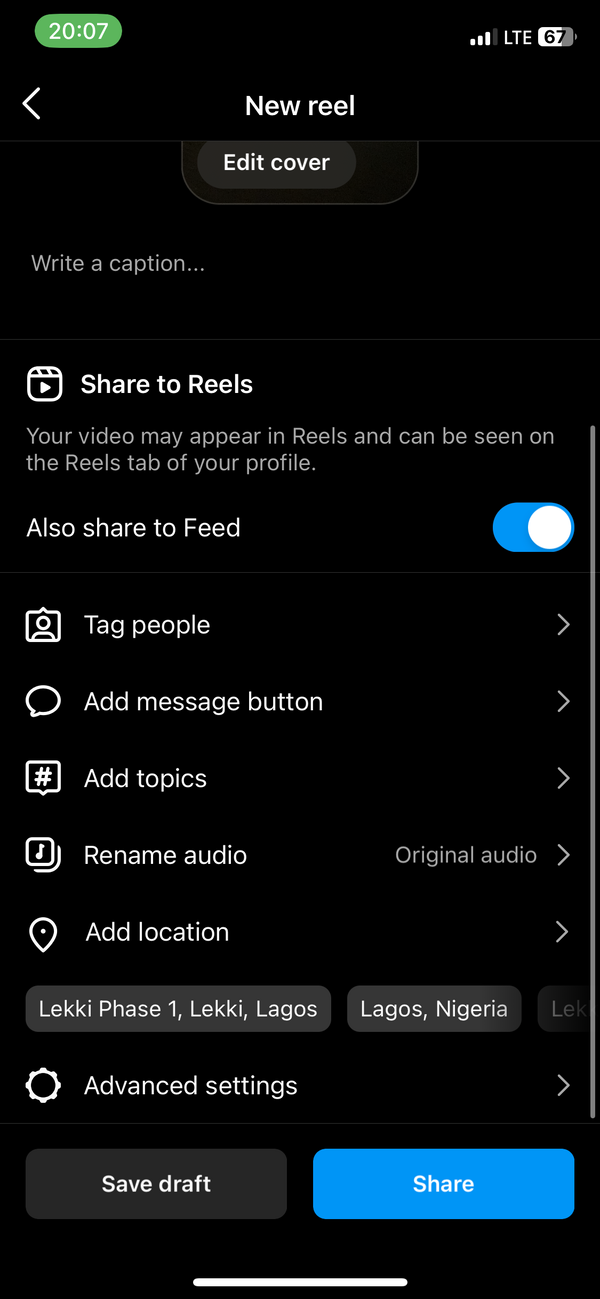The image displays a screenshot of a cell phone, showcasing the user interface for sharing a video to Instagram Reels. In the upper left corner, against a green background, the time is shown as 20:07. The upper right corner indicates a 67% battery level, LTE connectivity, and three bars of signal strength.

Central to the image, a black background presents the main interface titles: "New Reel," "Edit Cover," and "Write a Caption." Beneath these titles, a message reads: "Your video may appear in Reels and can be seen on the Reels tab of your profile." Below this, a toggle switch labeled "Also share to Feed" is turned on.

Several interactive options with right-arrow icons are available for users to further customize their post, including:
- Tag People
- Add Message Button
- Add Topics
- Rename Audio
- Original Audio
- Add Location

Additionally, three buttons listed as "leaky phase one," "leaky logos," and "logos Nigeria" are presented, along with an "Advanced Settings" option denoted by a circular gear wheel and a right-arrow icon for further settings.

At the very bottom of the screen, two buttons are visible: "Save Draft" and a prominently highlighted "Share" button in blue.

This detailed screenshot provides an informative view of the Instagram Reels sharing interface, highlighting the numerous customization options and settings available to the user.